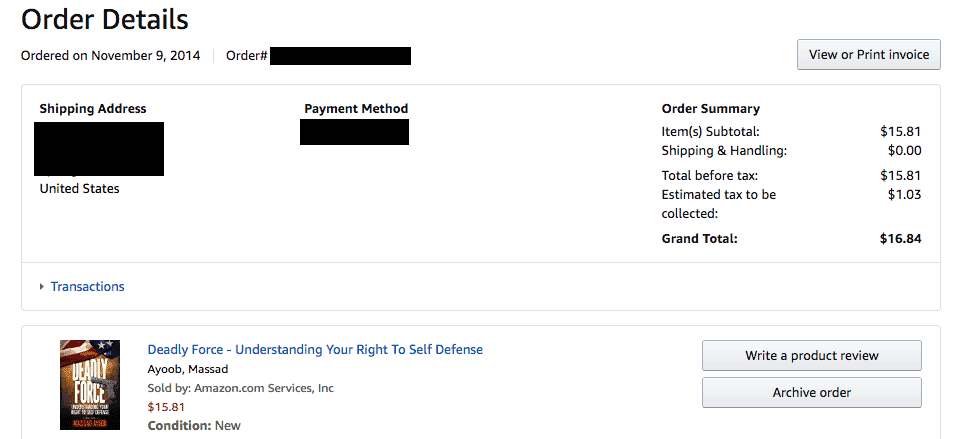**Detailed Caption:**

This image is a screenshot of an order details page from an e-commerce website. In the top left corner, the header reads "Order Details." Below that, it displays "Ordered on November 9, 2014" and "Order Number," with the actual order number blacked out for privacy. In the upper right corner, there is an option to "View or Print Invoice."

On the left side, under "Shipping Address," the actual address is obscured, but it's followed by "United States." Below this, it lists "Payment Method," which is similarly blacked out. 

The right column provides an "Order Summary," detailing:
- Items Subtotal: $15.81
- Shipping & Handling: $0.00
- Total before Tax: $15.81
- Estimated Tax to be Collected: $1.03
- Grand Total: $16.84

To the left, there is a small icon of the product, which appears to be a book cover. The cover features an American flag at the top and is titled "Deadly Force" with a revolver pictured partially over the title. The text beneath the title "Deadly Force" is too blurry to be legible, including the author’s name.

To the right of the book cover, details about the book are displayed:
- Title: "Deadly Force: Understanding Your Right to Self-Defense"
- Author: A.U. Massad
- Seller: Amazon.com Services, Inc.
- Price: $15.81
- Condition: New

To the far right, there are options for "Write a Product Review" and "Archive Order."